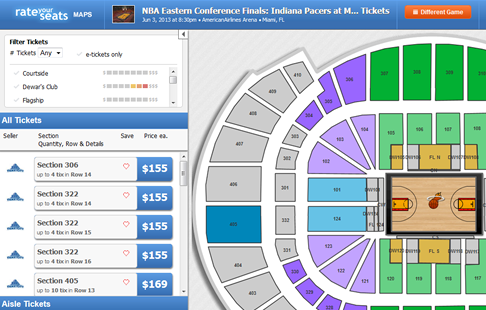This screenshot captures a web page for an NBA Eastern Conference Finals game between the Indiana Pacers and Miami Heat. The website's name appears in the upper left corner on a blue background with white text, featuring the prompt "Rate Your Seats." To the right, details of the event are listed, indicating the game is scheduled for June 3, 2013, at 8:30 PM at an arena in Miami, Florida. The text is quite small and somewhat blurry, but these details are discernible. In the upper right corner, there's an orange button labeled "Different Game." Below this, on the right side of the page, there is a detailed diagram of the seating sections surrounding a basketball court. The seats closest to the court are color-coded in green, lavender, and blue. Moving outward, the next level of seating is marked in dark green, purple, and gray. The topmost sections are predominantly gray, with the exception of a single block highlighted in teal.